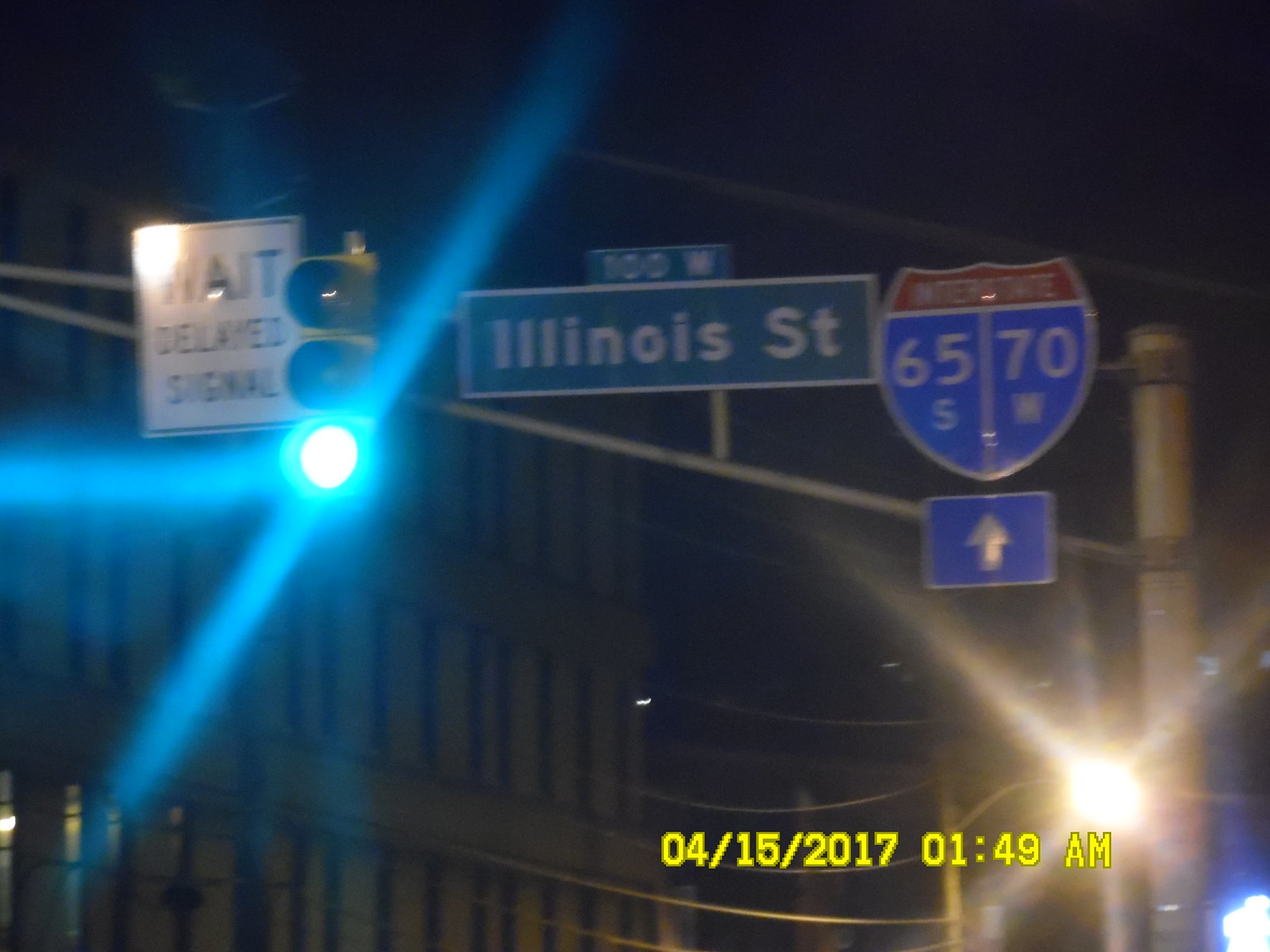The photograph, taken outdoors at night from a street, captures an urban scene under a dark sky with a building faintly visible in the background. In the lower right corner of the image, a bright yellow timestamp reads "4-15-2017, 1:49 AM." Central to the composition is a tall gray pole adorned with various street signs. 

Starting from the top left of the pole, a square white sign with black text reads "Wait Delayed Signal." Adjacent to it, a traffic light glows green. Below and to the right, there is a traditional green street sign with a white border; the upper section reads "100 West," and beneath it, "Illinois Street." Further to the right, there's a shield-shaped sign in red, white, and blue, indicating the interstate highways: "65 South" on the left and "70 West" on the right. Below this interstate sign is a blue rectangular sign featuring a silver arrow pointing upward, likely indicating a straight route. The building on the left side of the image has a facade with vertical lines, hinting at an urban setting.